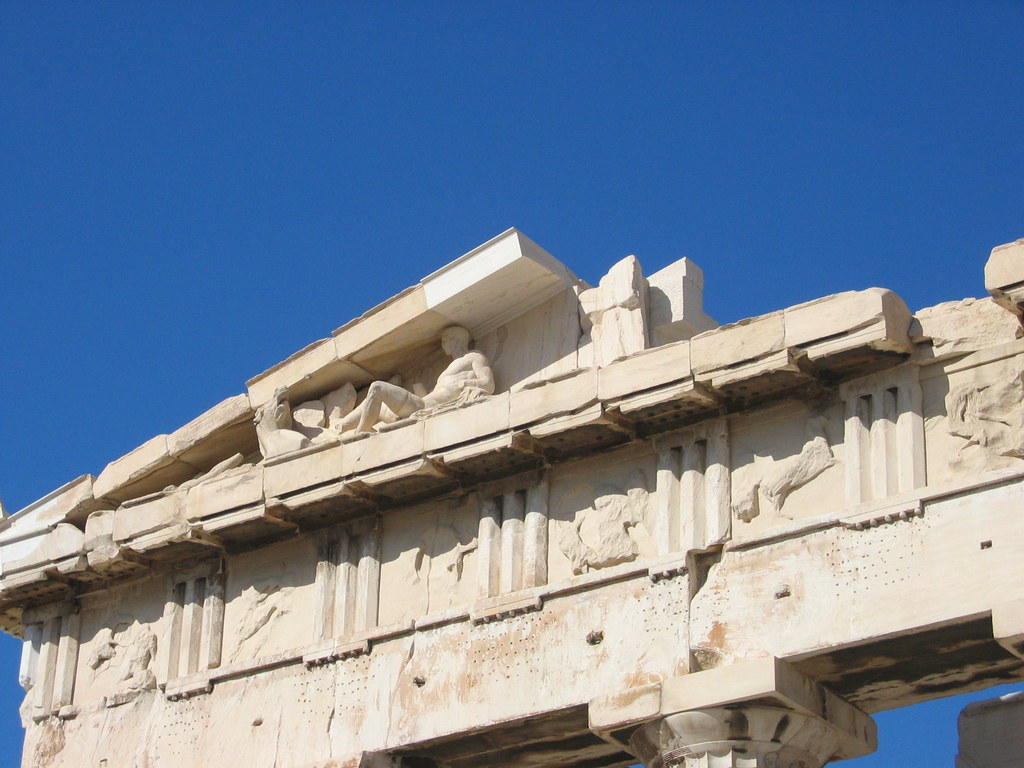The image is a detailed outdoor photograph capturing the ancient Roman-esque architecture of an old stone building made from white stone that displays multiple discolored, dirty spots in darker tan shades. The close-up focuses on the upper portion of the structure, revealing artistic carvings and reliefs that are somewhat deteriorated with age. Prominently, in the upper left portion of the image, there is a carved statue of a man in a reclining pose, propped up on his elbows, looking upwards. Above him, the remains of what might have been a roofline are visible, suggesting a triangular design that now appears broken or cut out. The structure as depicted is hundreds of years old and shows significant signs of wear. In the lower right corner, one can discern the tops of some pillars, hinting at the support for the building. The backdrop features a bright, cloudless blue sky, emphasizing the dilapidated yet grand majesty of the ancient stone edifice.